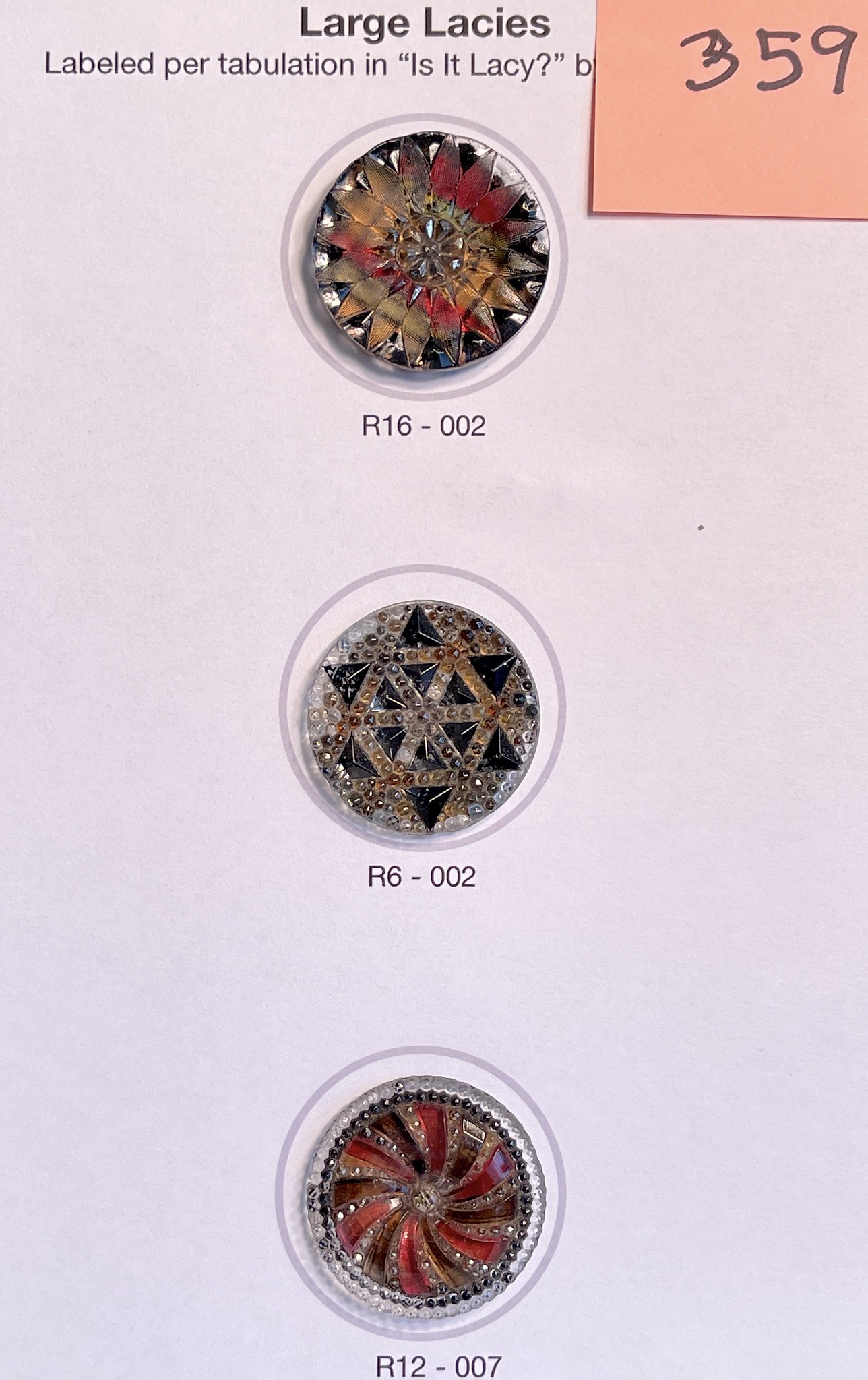In this detailed image set against a very light purple background, there are three circular ornaments arranged vertically in a row, each with intricate designs and labeled descriptions. At the top, in bold black letters, it reads "LARGE LACYS" followed by the phrase "LABEL PER TABULATION" in smaller, less clear text. An orange post-it note with the handwritten number "359" is positioned in the top right corner, partially obscuring the text. The topmost ornament looks like a star with dark red and orange hues, labeled "R16-002." The middle ornament features a star with fewer points, black edges, and adorned with beads, labeled "R6-002." The bottom ornament has a swirling design in a blend of red and brown colors and is labeled "R12-007." Together, the image presents a detailed and colorful display, potential indicative of jewelry or decorative items.